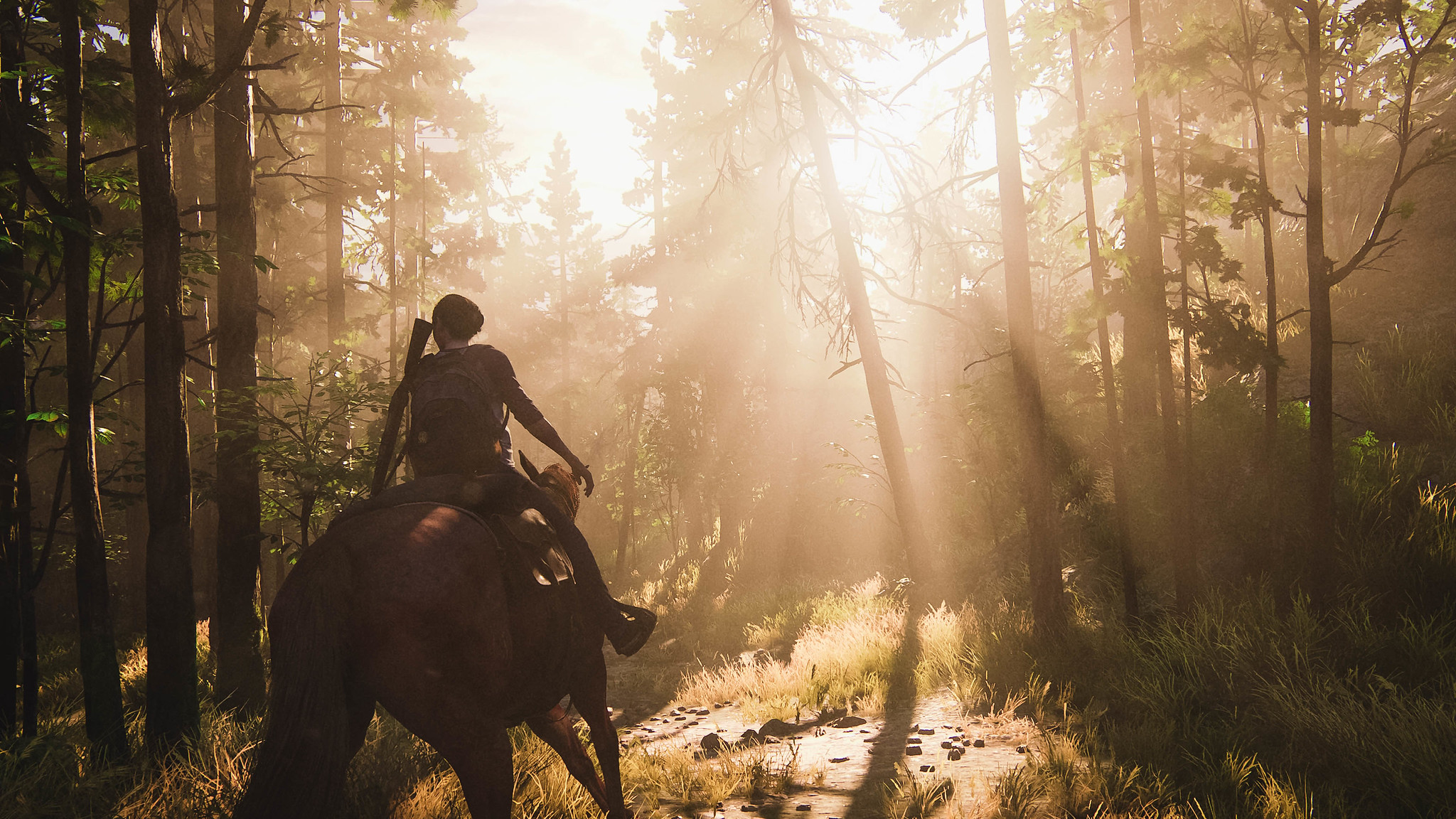The image appears to be from a video game, depicting a scene from a forest. A person, possibly a woman with her hair in a bun, is riding a horse and facing left. Both the rider and horse are viewed from behind. The rider has a backpack and a long-barreled gun slung over their left shoulder. The sun is shining brightly through the trees, casting rays of light onto the ground, which is a mix of grass, weeds, and bare dirt. The trees in the forest vary; some are evergreens with large trunks, while others are tall with thin trunks, and some lack leaves. The scene captures the serene atmosphere of riding through a sunlit forest, with light filtering through the high-reaching trees.